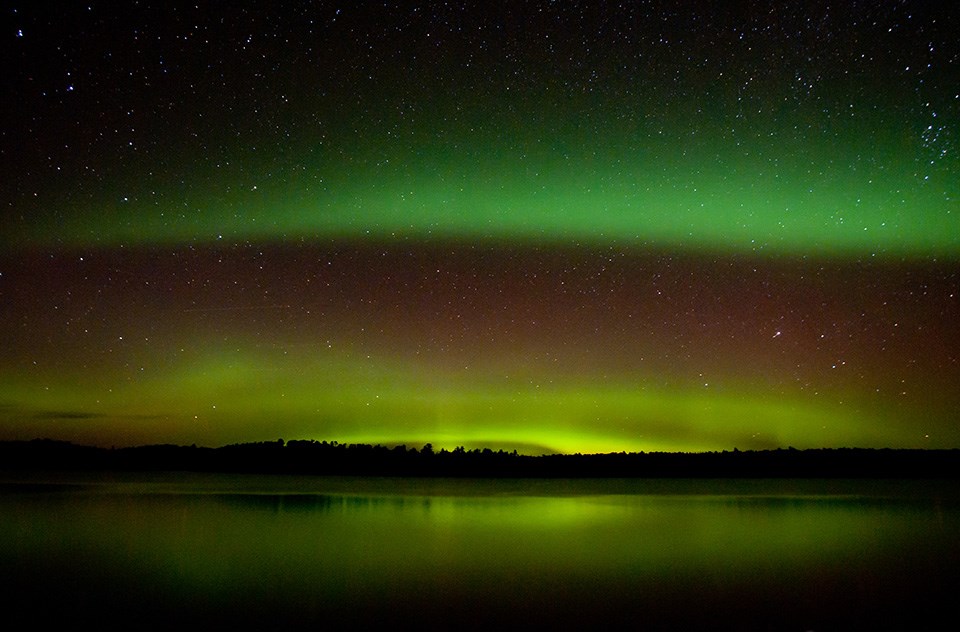This captivating nighttime photograph showcases the Northern Lights casting a mesmerizing green hue across the sky. The scene is dominated by the vibrant auroras, which paint the sky in bands of green, yellow, and chartreuse. These lights stretch majestically across the horizon, reflecting on the serene, calm surface of a large lake in the foreground. The reflection of the auroras on the lake creates a mesmerizing mirror effect, enhancing the ethereal quality of the scene. Silhouetted against this spectacle are low hills densely covered with trees, adding depth and contrast to the image. Above the bands of colorful auroras, a vast expanse of purple-blue-black sky is dotted with countless stars, creating a tapestry of celestial beauty. The scene is devoid of any signs of civilization, emphasizing the untouched, natural purity of this breathtaking moment. The overall effect is one of tranquil, shimmering brilliance, capturing the majestic beauty of the Northern Lights in a professional-quality landscape photograph.